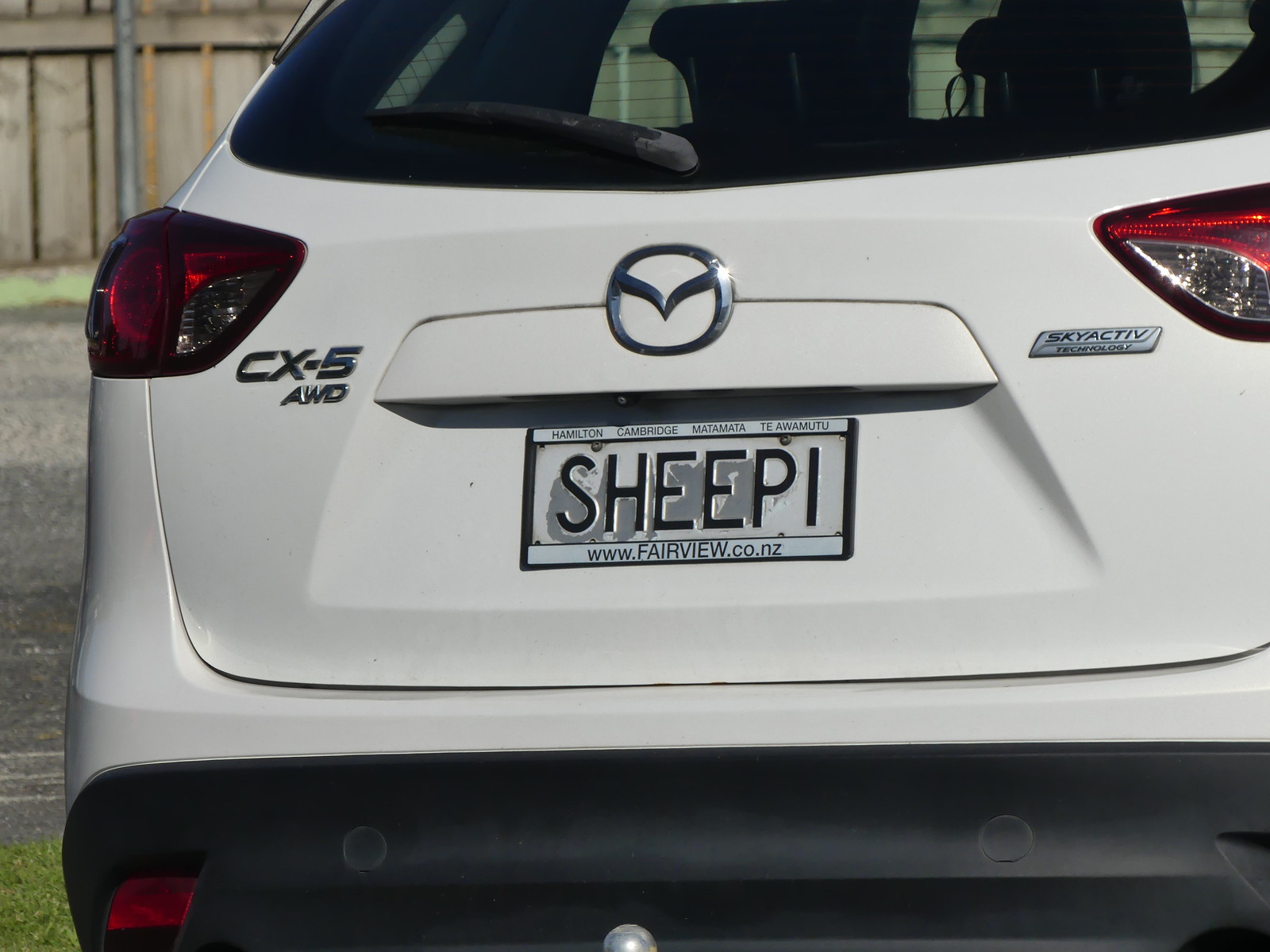This image captures the back of a white Mazda CX-5 SUV, prominently showcasing its features. The vehicle displays a silver "CX-5" badge on the left and "AWD" indicating it has all-wheel drive capabilities. On the right, it features the "SKYACTIV" badge, noted for its unique spelling without an "E" at the end, a stylistic touch that signifies Mazda's advanced technology. The custom license plate reads "SHEEPY" in black letters on a white background, accompanied by a URL, www.fairview.co.nz, suggesting the vehicle may be from New Zealand. The SUV's rear end is marked by red brake lights with white backup lights below and a black bumper with a visible silver hitch. The backdrop includes a light brown wooden fence, green grass, and a gray road, providing a setting that hints at a residential or suburban area.